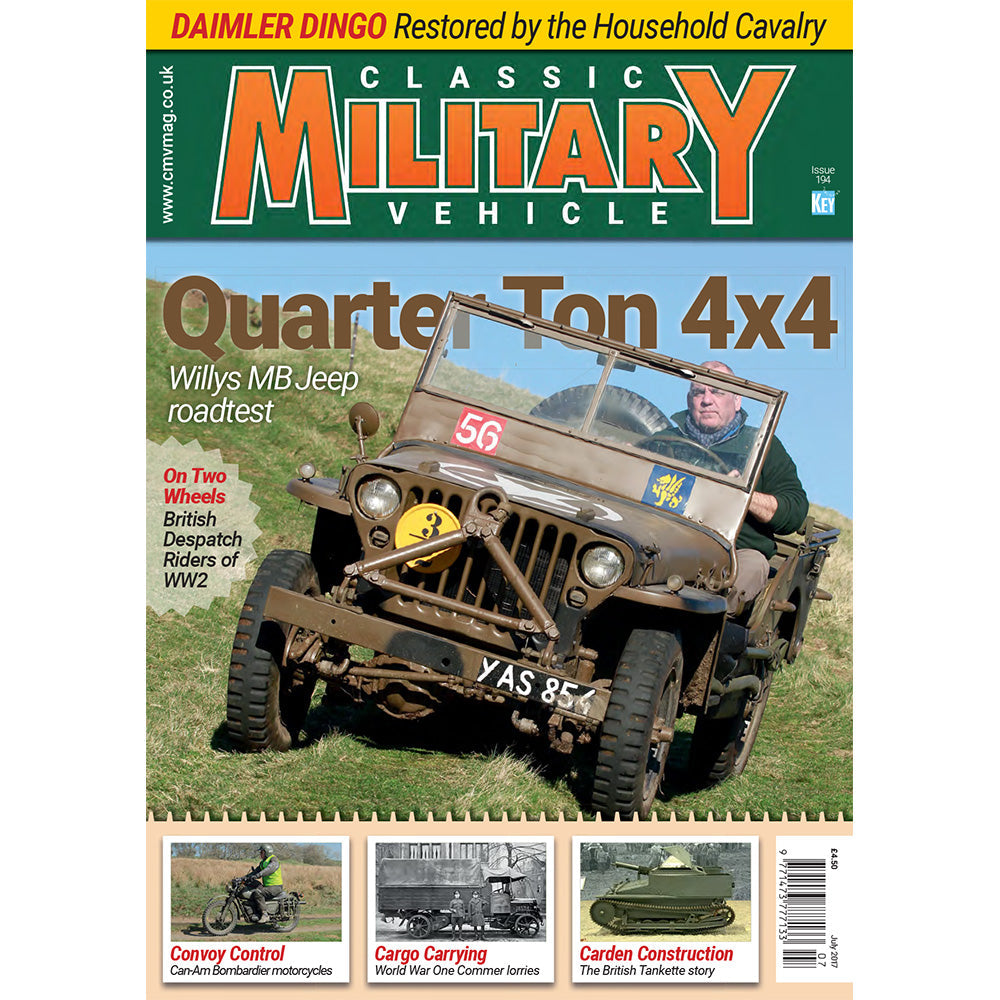This captivating magazine cover, titled "Classic Military Vehicle," prominently features a central image of a man driving a quarter-ton 4x4 jeep, reminiscent of a military or army vehicle. Facing the viewer, the jeep's dark brown exterior is clearly visible, showcasing its circular headlights and distinctive black and brown grille. The driver is dressed in a green sweater and gray pants, navigating the jeep up a grassy hill.

At the bottom of the cover are several detailed side-profile images of other military vehicles. One shows a man riding a motorcycle, another features a large cargo vehicle, and the last image highlights a green tank. Each vehicle is meticulously depicted, adding to the magazine’s comprehensive exploration of classic military machinery.